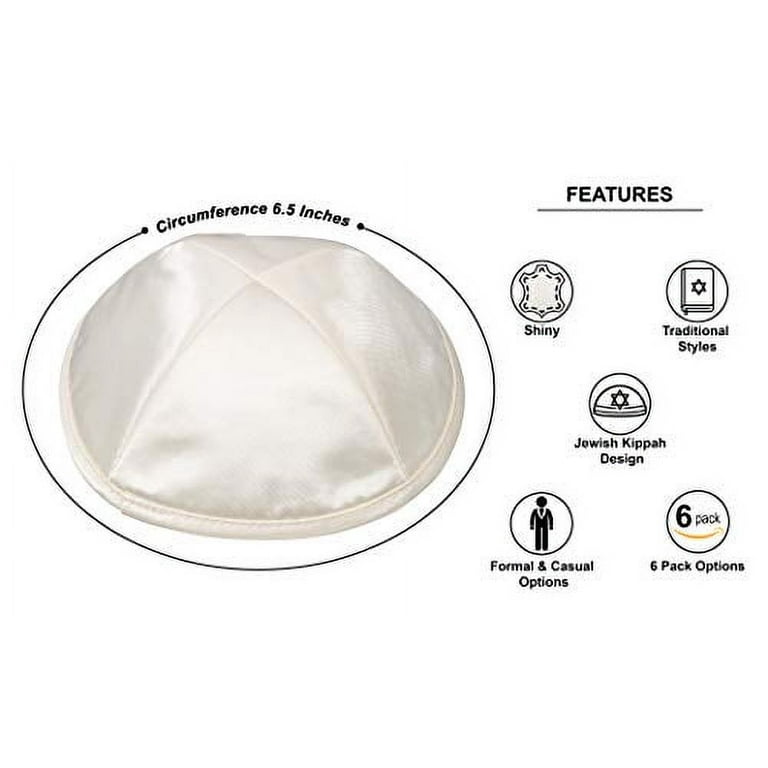The image is an advertisement for a traditional Jewish yarmulke, also known as a kippah. The featured kippah is white with a satin finish, showcasing a subtle sheen. The primary focus is on the kippah's detailed quilting, forming an 'X' on the top, with a line encircling it and a clear indication of its circumference, measuring 6.5 inches. To the right, bold black letters read "FEATURES" with a line beneath it, and several circles present individual icons for each feature. One circle highlights the kippah's shiny texture, while another emphasizes its traditional style with a Star of David atop a book, presumably a Torah. Additional circles showcase the kippah's Jewish design, another Star of David, and options for both formal and casual wear indicated by a silhouette figure. Finally, there is a circle highlighting a six-pack purchase option, marked with a yellow arrow reminiscent of the Amazon logo.